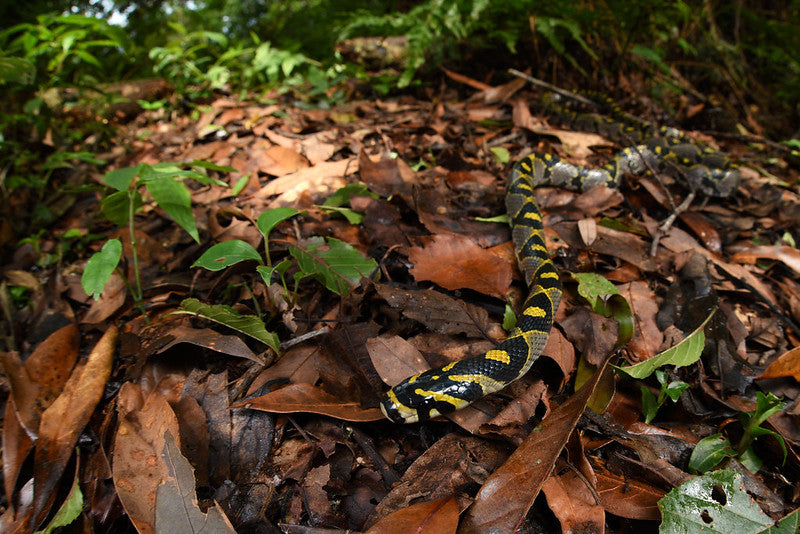The photograph captures a vibrant, detailed scene in a sunlit forest or jungle area. The ground is densely covered with wilted, brown dead leaves interspersed with small green plants and foliage sprouting from the earth. Dominating the right-hand side of the image, a very long snake—presumably over six feet—slithers gracefully from the top right to the middle bottom of the frame. The snake's intricate scale pattern features striking black and yellow diamond shapes, suggesting it could be poisonous. This focused nature photography highlights the snake as the main subject, with the rich, leafy background contributing to the lush, realistic ambiance reminiscent of a nature textbook.